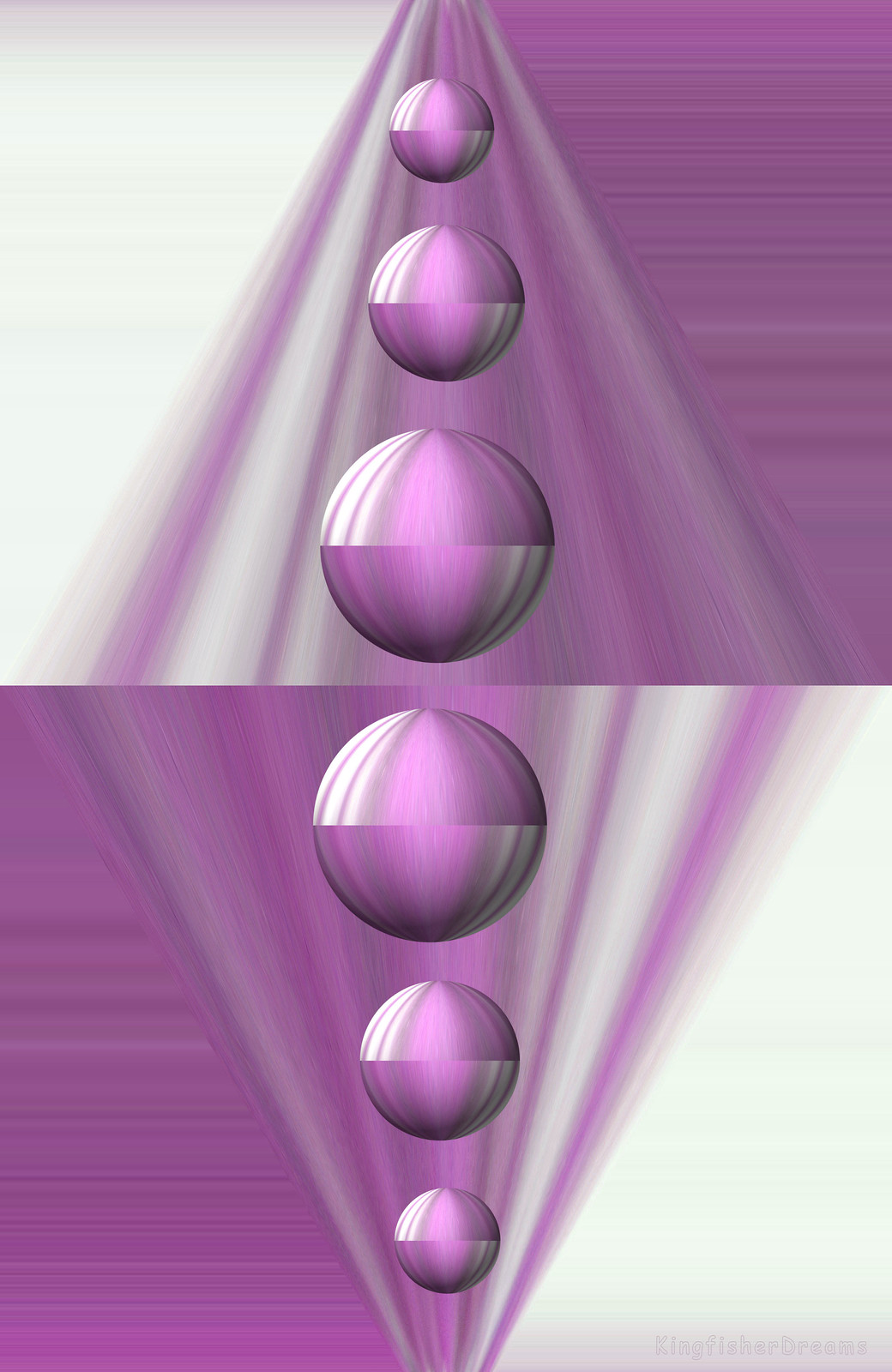The image is an abstract, possibly computer-generated artwork featuring a complex interplay of purple and white elements. A prominent diamond shape, formed by blurry, abstract purple lines, dominates the center. Running vertically through the diamond are six highly reflective purple spheres, arranged in a gradient of sizes—smallest at the top and bottom, medium in the vicinity, and the largest in the center.

The image is divided into four quadrants, adding to its intriguing symmetry. The top left and bottom right quadrants have a contrasting white background, while the top right and bottom left quadrants share the same purple backdrop. The top and bottom halves of the image mirror each other but are flipped 180 degrees. This creates a sense of mirrored asymmetry where the left bottom and top right corners are both purple, and the top left and bottom right corners are white.

Additionally, purple and white diagonal stripes are present in the white background areas, further enhancing the abstract quality of the artwork. The image's design gives a perspective effect, where lines taper from a wider base to a narrower point at the top in the upper half, and vice versa in the lower half. This creates a dynamic visual pathway that seems to invite the viewer's gaze to travel along the contours of this intriguing piece.